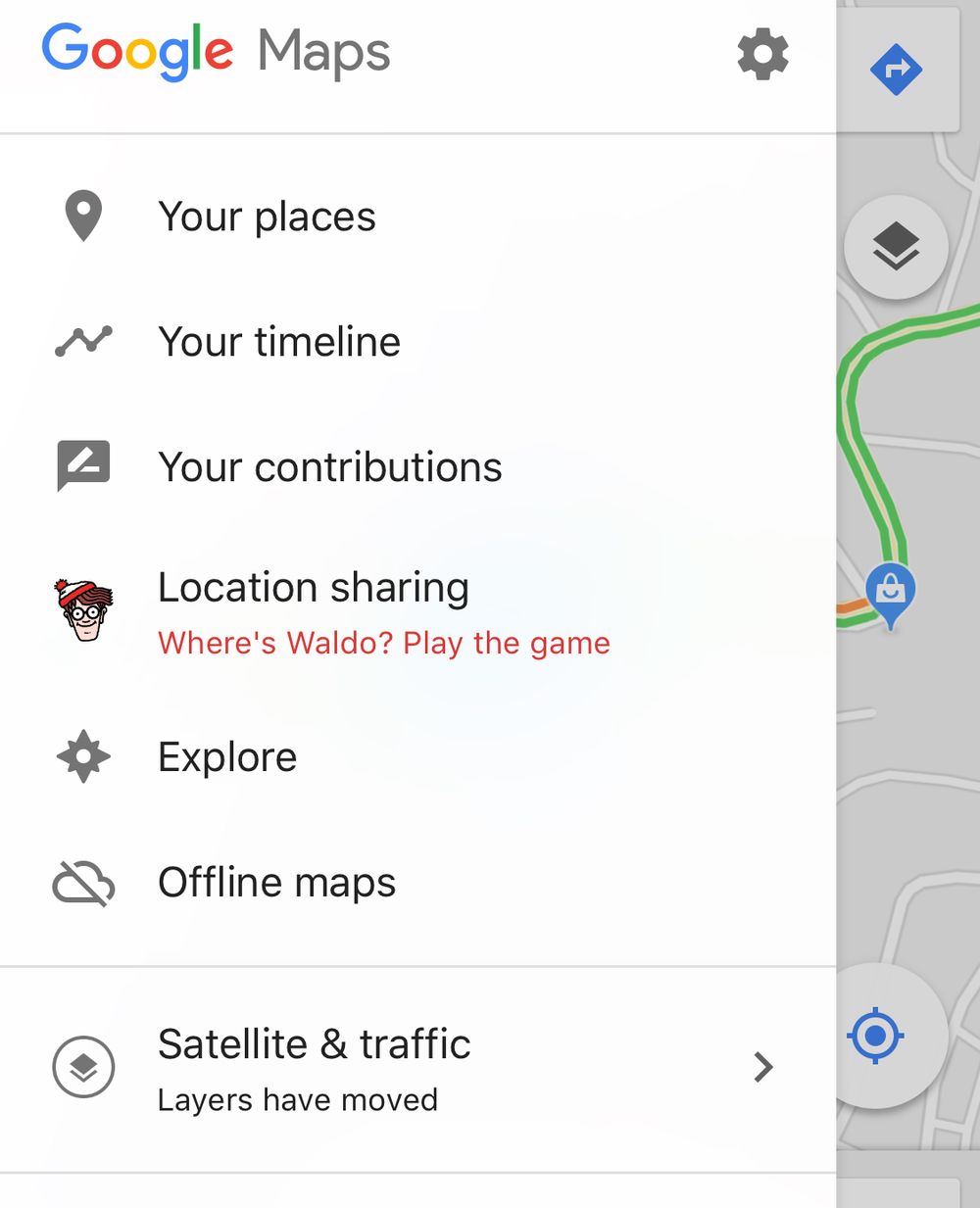A screenshot, presumably from a phone, showcases a section of the Google Maps interface. At the very top against a white background, there is the multicolored Google logo, followed by the gray word "Maps" and concluding with a gray settings icon on the far right. Below this header, separated by a thin gray horizontal line, lies a menu with various features.

From left to right, the gray pin icon labeled "Your Places" is followed by a black zigzag line with four points labeled "Your Timeline." Next, a gray speech bubble containing a pen or pencil icon leads to the "Your Contributions" label.

Further down, an illustration of Waldo from the "Where's Waldo" series, characterized by his red, brown, and Caucasian features, is accompanied by the label "Location Sharing: Where's Waldo - Play the Game" in bold red text.

Below this, the menu continues with the word "Explore" next to a compass point icon, "Offline Maps" accompanied by a cloud icon with a diagonal line through it, and "Satellite and Traffic" next to a gray circle containing two overlaid squares, indicating the layers menu. To the right of this section is a gray right-facing arrow.

In the background of this window, glimpses of the Google Maps screen can be observed. Prominently visible on the upper right is a blue diamond shape with a white right arrow inside, amidst green curving lines against a gray background. Additionally, a blue pin with a white shopping bag icon is centrally located on a highlighted roadway. Towards the bottom right, there is a white circle featuring a compass point icon.